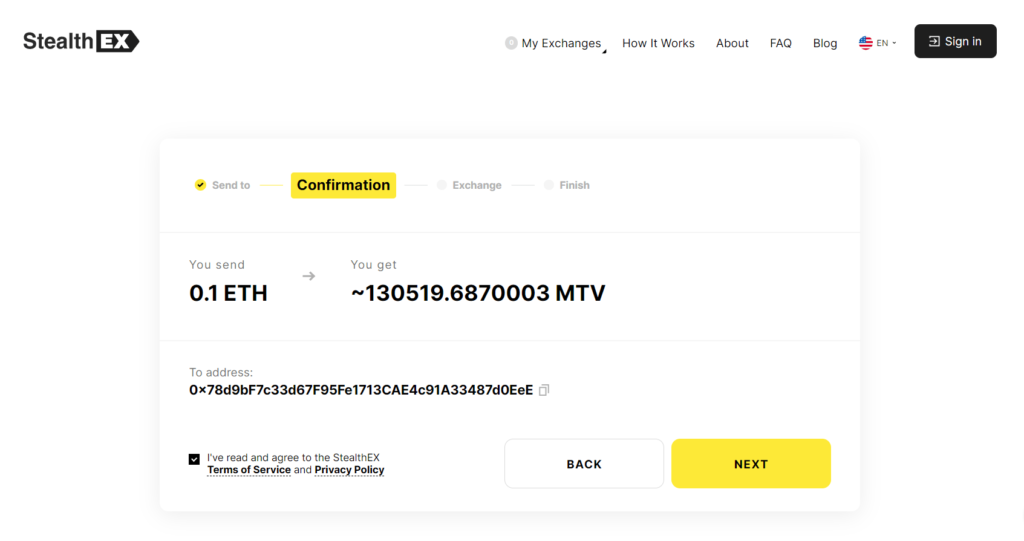This is an image of a confirmation screenshot from a computer interface. In the top-left corner, the title "Stealth EX" is displayed with "EX" in a rightward-pointing black arrow. On the right-hand side of the screen, there are several navigational tabs available: "My Exchanges," "How It Works," "About," "FAQ," and "Blog." Additionally, there is an option for selecting the language, currently set to English, indicated by "EN" and accompanied by an American flag. A black pill-shaped button labeled "Sign In" is also visible.

Below this header section, a white box outlines the steps of the transaction process. The first step, "Send To" has been completed, marked by a yellow circle with a black checkmark. The current step, "Confirmation," is highlighted in a yellow box. The subsequent steps, "Exchange" and "Finished," are also listed but not yet highlighted. 

Details of the transaction are provided beneath the step indicators: it shows that 0.1 ETH has been sent and, in return, 130,519.6870003 MTV will be received. The recipient's address is displayed as a long string of alphanumeric characters. 

Towards the bottom of the screen, there is a checkbox on the left confirming the agreement to the Terms of Service and Privacy Policy. On the right, two pill-shaped buttons are visible: a white one labeled "Back" and a yellow one labeled "Next."